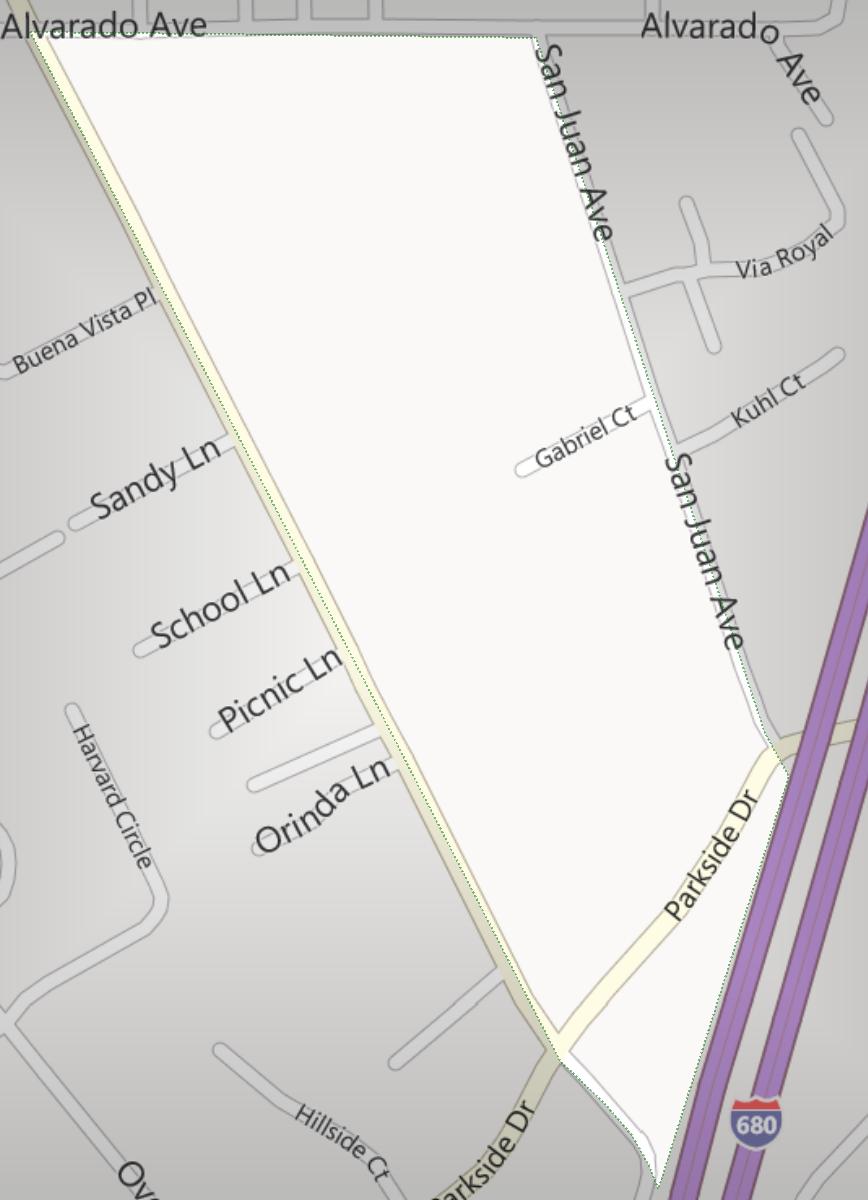The map displayed is of an unidentified area, with a prominent, unlabeled white strip running diagonally from the top left to the lower right corner, possibly highlighted but not indicative of a river. The uppermost part of the map is spanned by Alvarado Avenue, which takes a diagonal downturn at the top right corner. San Juan Avenue branches downward at an angle from Alvarado Avenue. Two primary roads emanate from Alvarado Avenue, with one remaining unnamed. Along San Juan Avenue, you'll find Valle Royal, Gabriel Court, and Cool Court, while Parkside Drive intersects both San Juan Avenue and the unnamed street. 

From the upper left of the map down along the unnamed street are Buena Vista Place, Sandy Lane, School Lane, Picnic Lane, and Orinda Lane. Near the lower section of the map, Hillside Court extends from Parkside Drive. In the lower left corner, a partially visible diagonal street ending in "OV" is present, along with Harvard Circle branching off from it.